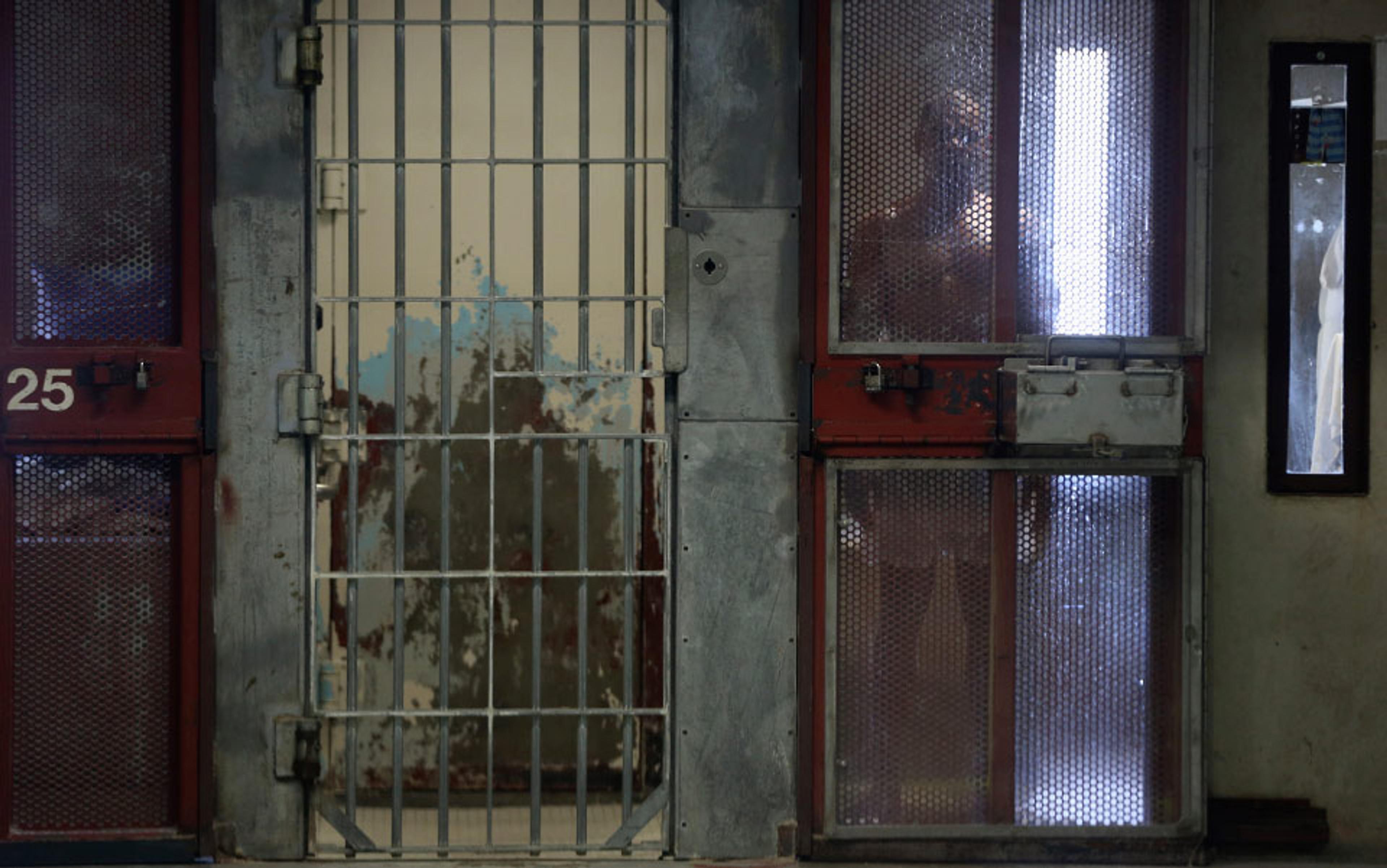The image depicts a bleak and desolate prison setting. The left side of the scene is dominated by a gated red screen door marked with the number 25. This door is securely padlocked, emphasizing confinement. To the right of this is another barred door with a metal keyhole and three hinges, reinforcing the grim atmosphere. Further to the right, a man stands behind a textured glass door that also has a central opening, likely for passing food into the cell without compromising security. This door is likewise padlocked, contributing to the forbidding environment. The man, who appears somewhat blurry through the textured glass, is standing with his arms at his sides, possibly unclothed. The background of his cell is barely lit by a window, the main source of light in the otherwise dark and drab room. The wall behind him has peeling paint in various shades of gray and blue, adding to the depressing and neglected ambiance. To the far right, a tall, narrow window framed in black offers another slight glimpse into the man's cell, enhancing the overall sense of isolation and confinement.